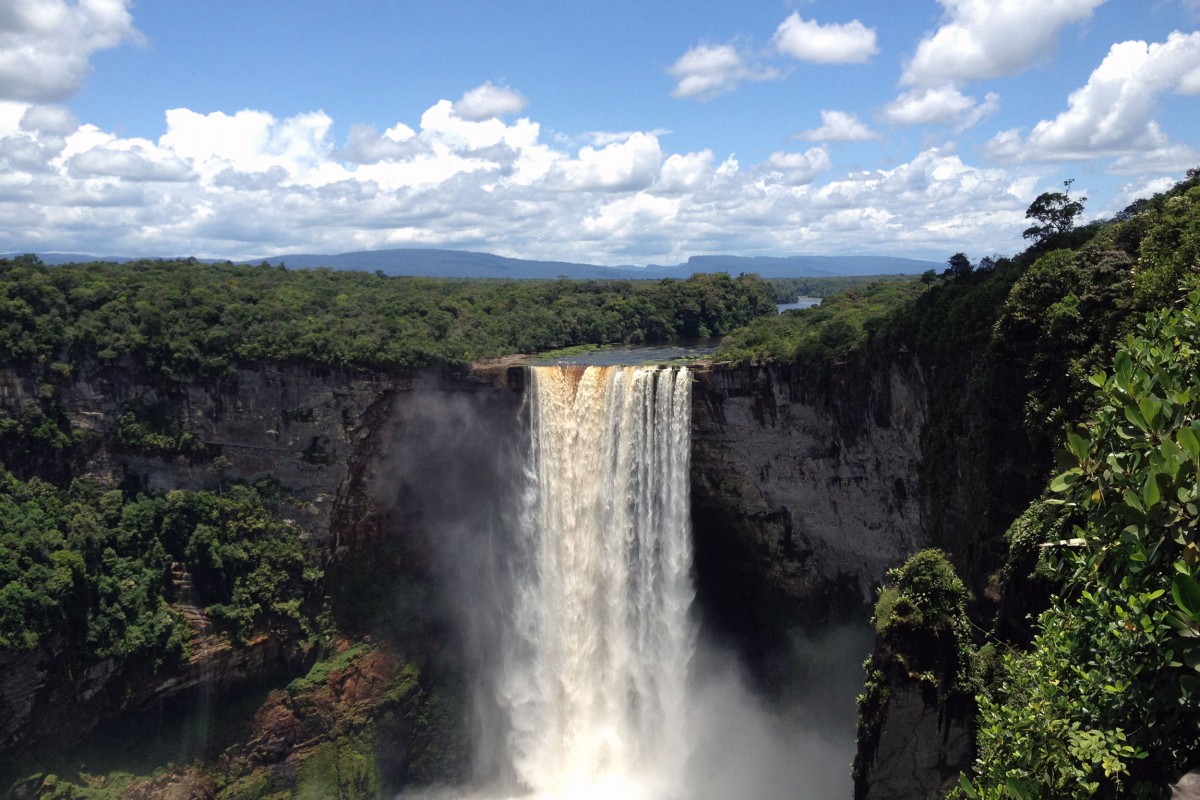The image captures a stunning, large waterfall situated in a picturesque natural setting. The waterfall dominates the center of the photograph, cascading down towards the viewer with a powerful rush that churns up a mist. It is a bright and clear day, with fluffy clouds dotting the blue sky, which takes up the top half of the photo. Surrounding the waterfall, the landscape features dark gray to black rock cliffs, lush green vegetation, and distant mountain ranges. The river feeding the waterfall has a slight muddy brown tinge, possibly from sediments, adding a touch of earthiness to the scene. The photograph is taken from an aerial viewpoint, providing a full, breathtaking view of the falls and the verdant treetops below. The entire scene exudes a sense of serene beauty, making it a likely popular outdoor tourist attraction.